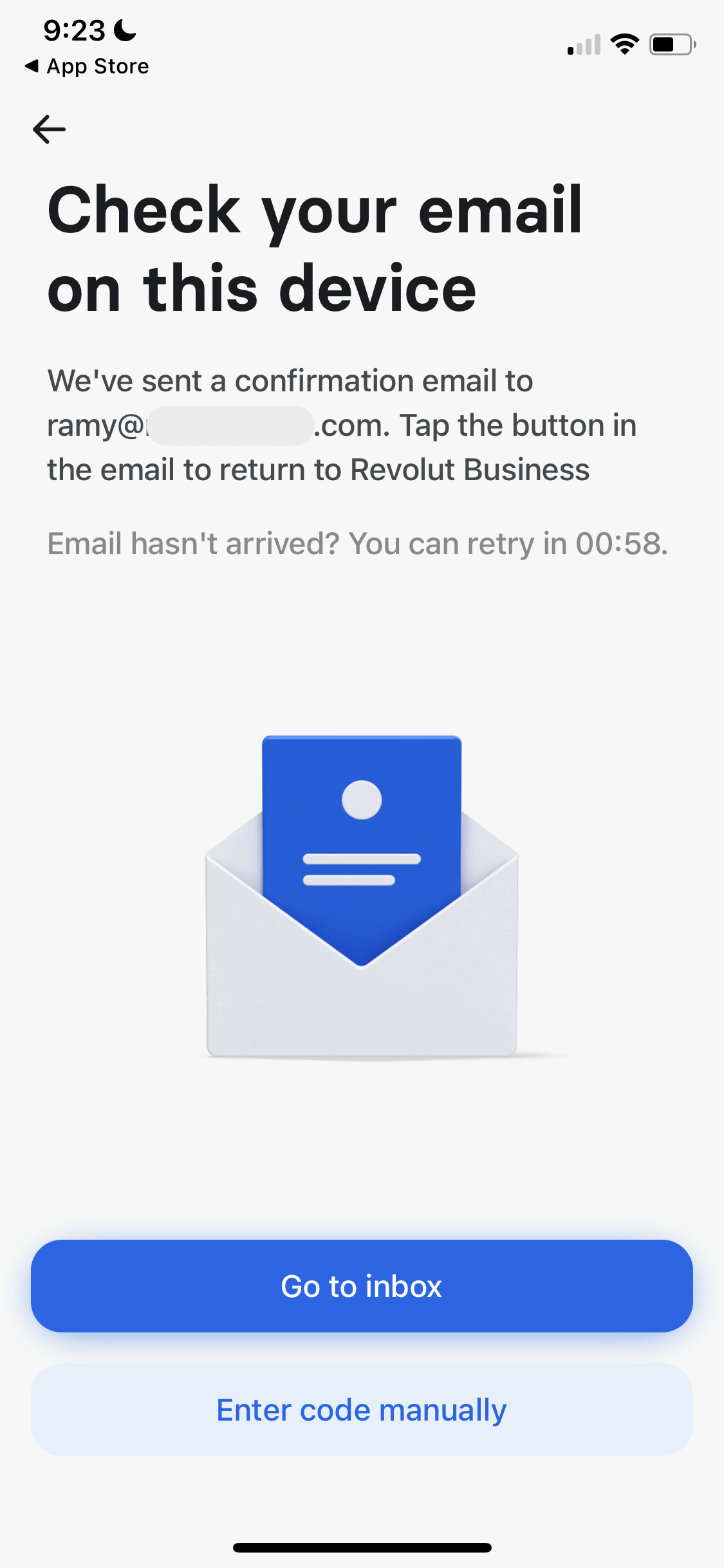The image is a screenshot of an iPhone screen displaying a confirmation message from Revolt Business. The prominent message reads: "Check your email on this device. We've sent a confirmation email to ramy [partially obscured] dot com. Tap the button in the email to return to Revolt Business." There is an additional note stating, "Email hasn't arrived? You can reply in 00:58," indicating a countdown of 58 seconds. Below this, there is a visual of a mail icon with a blue letter emerging from it. Two blue buttons follow: one that says "Go to Inbox" and a lighter blue one that says "Enter Code Manually." At the top of the screen, the time is displayed as 9:23, accompanied by a moon icon to the right, representing the Do Not Disturb mode. On the left, the status bar shows cellular service strength, Wi-Fi connectivity, and the battery percentage.